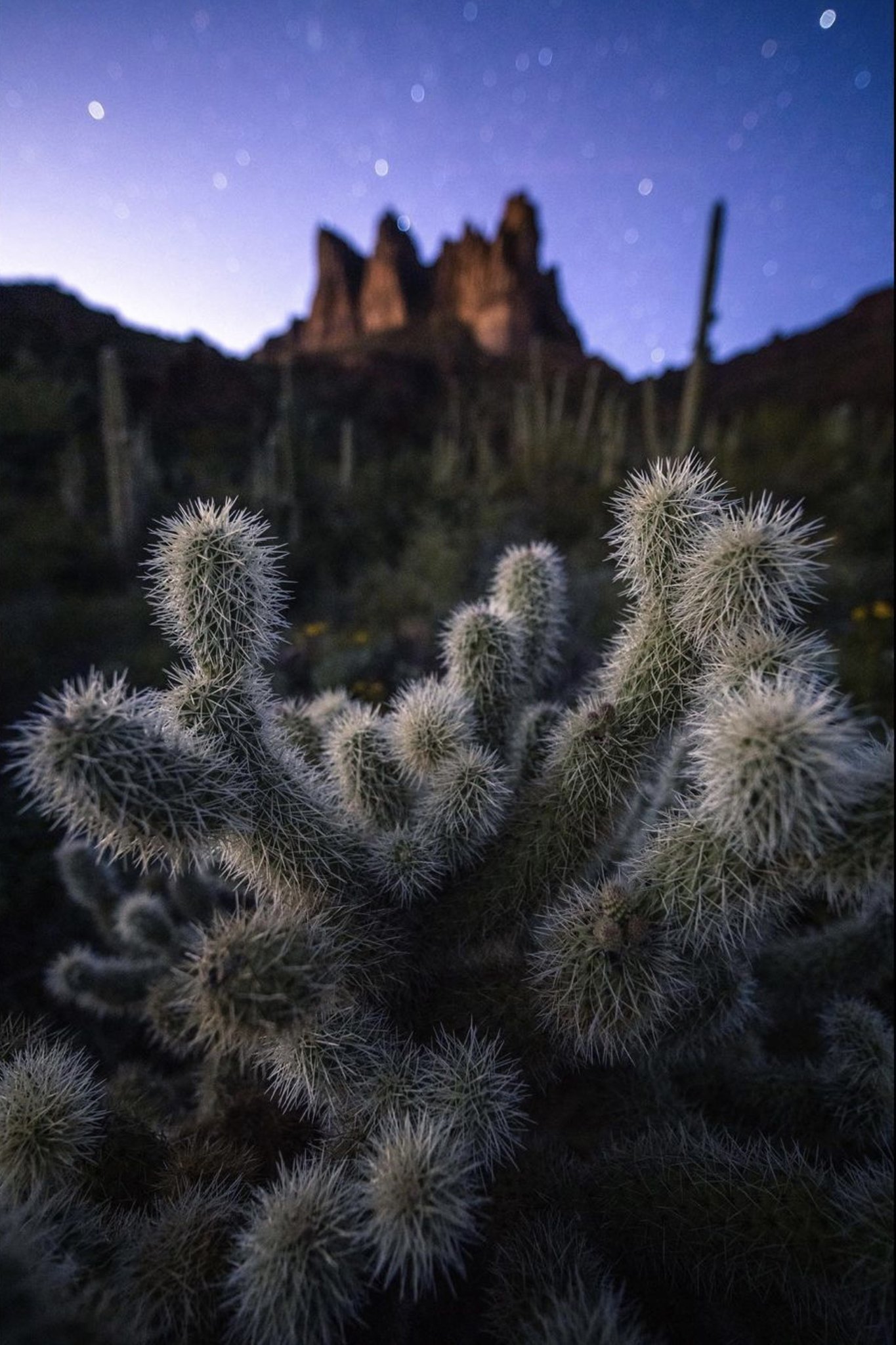This photograph captures a vibrant desert scene at dusk, teeming with cacti and accented by a dramatic landscape. In the foreground, a prominent green cactus with thick, curving stems densely populated with sharp, white thorns dominates the lower half of the image. Surrounding vegetation, including scrub and possibly yellow flowers, adds to the lushness of the scene. The background reveals a towering, craggy rock formation under a setting sun, its brown surface still illuminated by the last rays of daylight. The sky transitions from a dark blue to a vibrant purple near the horizon, punctuated by emerging stars that appear like tiny snowflakes, enhancing the twilight atmosphere. Tall cacti in the distance, their green stems blurry yet recognizable, add depth to this richly detailed desert landscape.